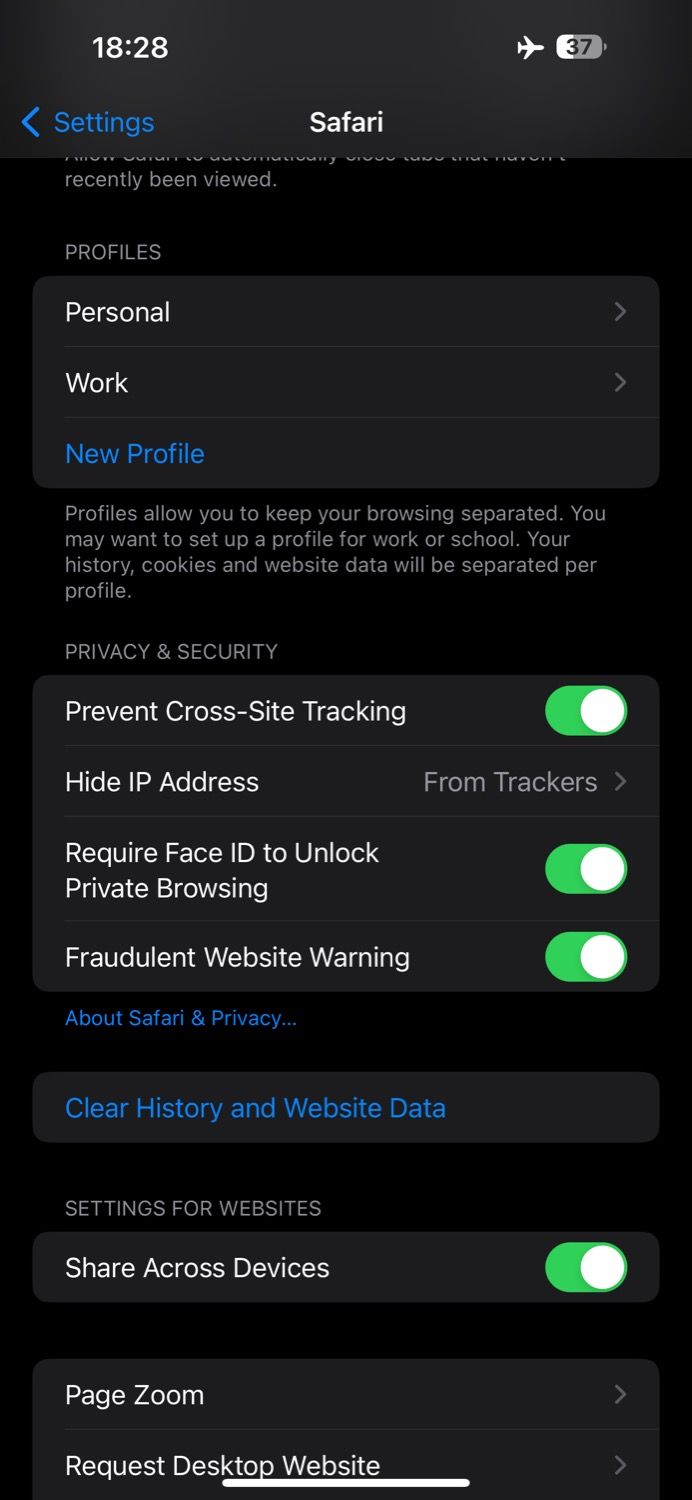The image depicts the settings page of an iPhone, focusing on the Safari browser settings. The screenshot was taken at 18:28 (6:28 PM) with the device in airplane mode, showing a 37% battery level.

At the top left, there's a back arrow with a blue hue, labeled "Settings," indicating that tapping it will return you to the main settings menu. The screen prominently labels the section as "Safari," under which various personal settings are displayed.

The settings page includes:
- **Profiles**:
  - *Personal*: An arrow to the right suggests additional options.
  - *Work*: An arrow to the right suggests additional options.
  - *New Profile*: A detailed explanation states, “Profiles allow you to keep your browsing separated. You may want to set up a profile for work or school. Your history, cookies, and website data will be separated per profile.”

- **Privacy & Security Settings**:
  - *Prevent Cross-Site Tracking*: Enabled.
  - *Hide IP Address from Trackers*: An arrow indicates more options.
  - *Require Face ID to Unlock Private Browsing*: Enabled.
  - *Fraudulent Website Warning*: Enabled (indicated by a white button slid to the right with a green background).
  - An option for "About Safari & Privacy."

- **Clear History and Website Data**: A dedicated heading for this action.

- **Websites**:
  - *Share Across Devices*: Enabled.
  - *Page Zoom*: Options available.
  - *Request Desktop Website*: Options available.

The background of the settings page is black, creating a high contrast for easy readability of the text and settings options.